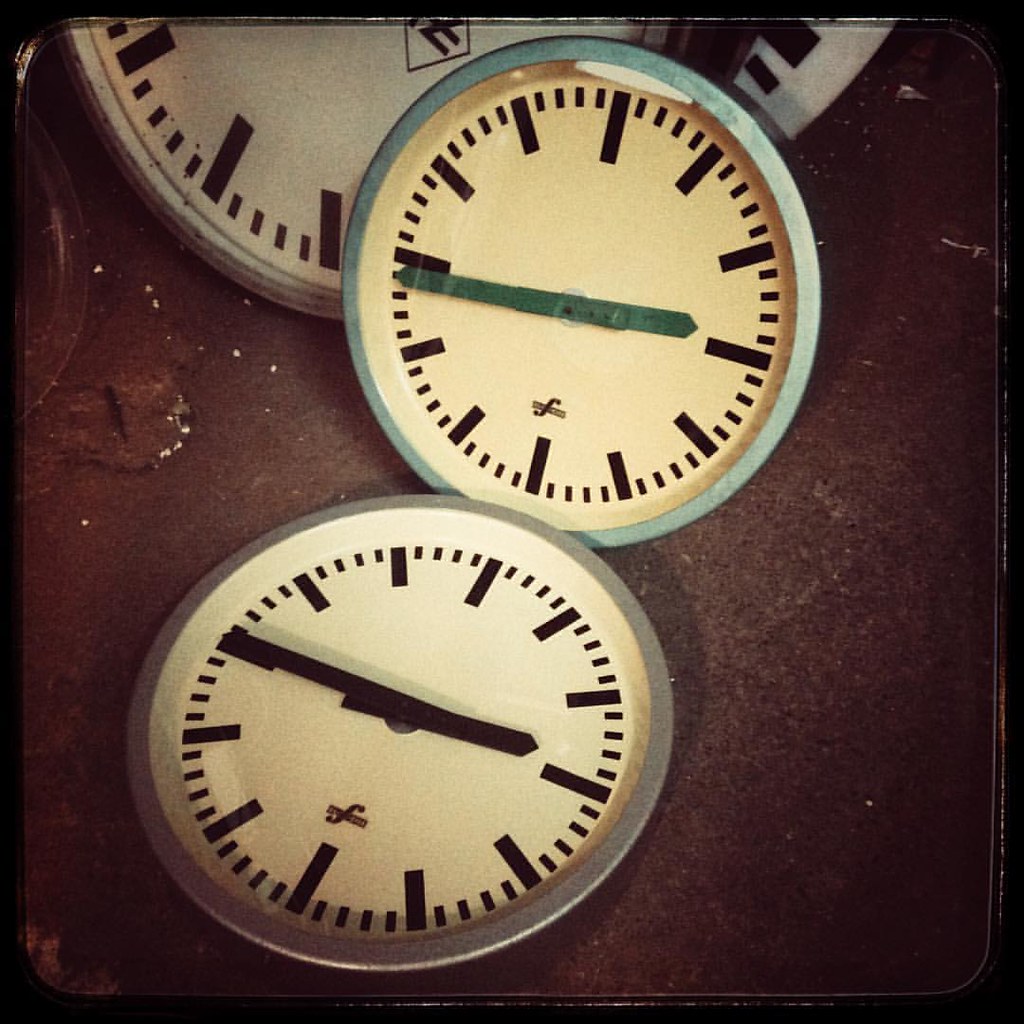The image showcases multiple small watch dials that appear to have been meticulously removed from their original watch settings. There are two fully visible dials and one partially obscured by the overlapping dials. Despite the overlap, the visibility of each dial is largely maintained. Each dial is circular, encased in a metallic frame. One of the fully visible dials features black hour and minute markers, while the other has green hour and minute markers. Notably, the markers on both dials are linear rather than numerical, giving them a unique appearance. The background of the dials is plain white, and the surface on which they rest appears to be glass, perhaps part of a microscope or another transparent, reflective surface.